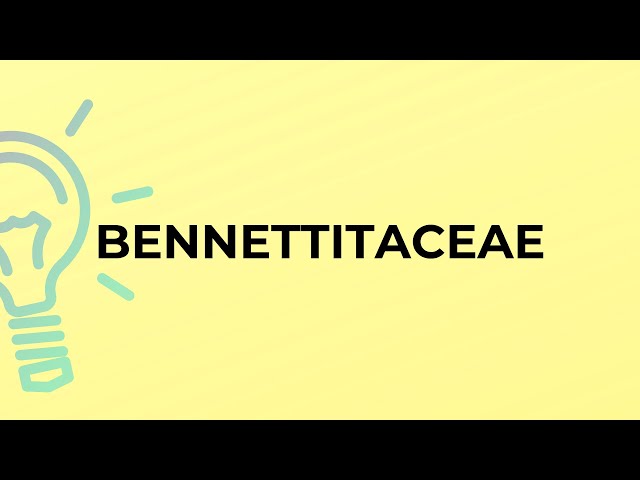The image features a computer-generated graphic resembling a logo. It consists of a bright yellow rectangle with thick black horizontal bands at both the top and bottom. Dominating the central part of the image is a large, light blue outline of a light bulb situated on the middle left. The light bulb has lines radiating from it, indicating it is illuminated. To the right of the light bulb, centered within the yellow background, is the word "BENNETTITACEAE" written in bold, capital letters. The layout is designed with the text running vertically down the center, with no other graphics present.